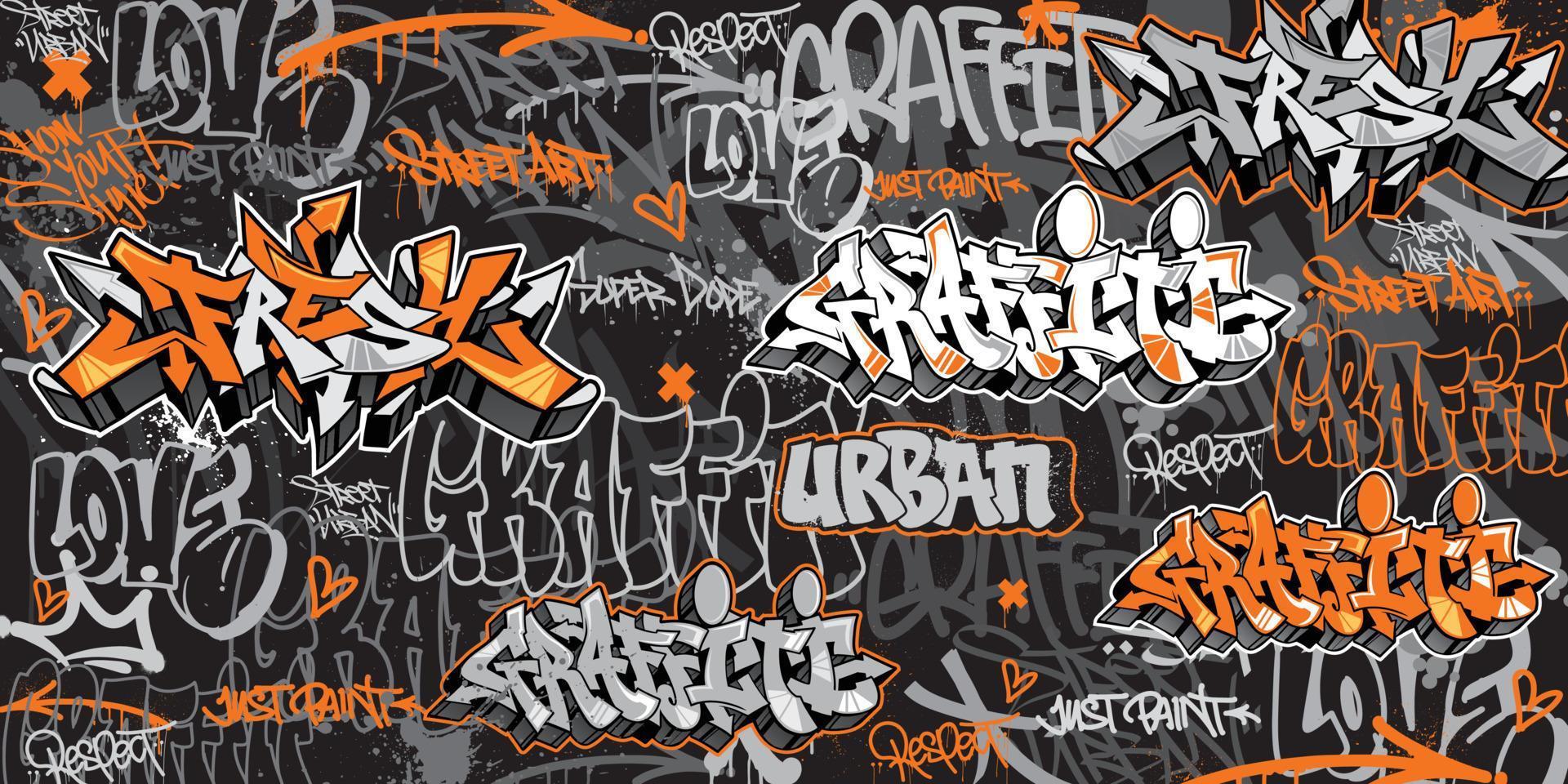The image is a digitally rendered, rectangular canvas filled with intricate graffiti. The base color of the wall is a blend of black and gray, overlaid with a vivid array of text in white, orange, and gray, with black accents. The most prominent words are "LOVE" and "GRAFFITI," repeated multiple times in various graffiti font styles. "LOVE" is often seen in distinctive gray bubble lettering, while "GRAFFITI" appears in both orange and gray, as well as in the same bubble font. Near the top left corner, the word "FRESH" stands out in a mix of orange and gray with detailed arrow embellishments. Additional words like "respect," "urban," "just paint," and "street art" are scattered across the image in smaller fonts. The graffiti also includes elements like hearts, arrows, X's, and a crown at the bottom left. The complex layering and diverse font styles lend a dynamic and three-dimensional feel to the artwork, making it a vibrant, decorative piece suitable for digital backgrounds or website aesthetics.